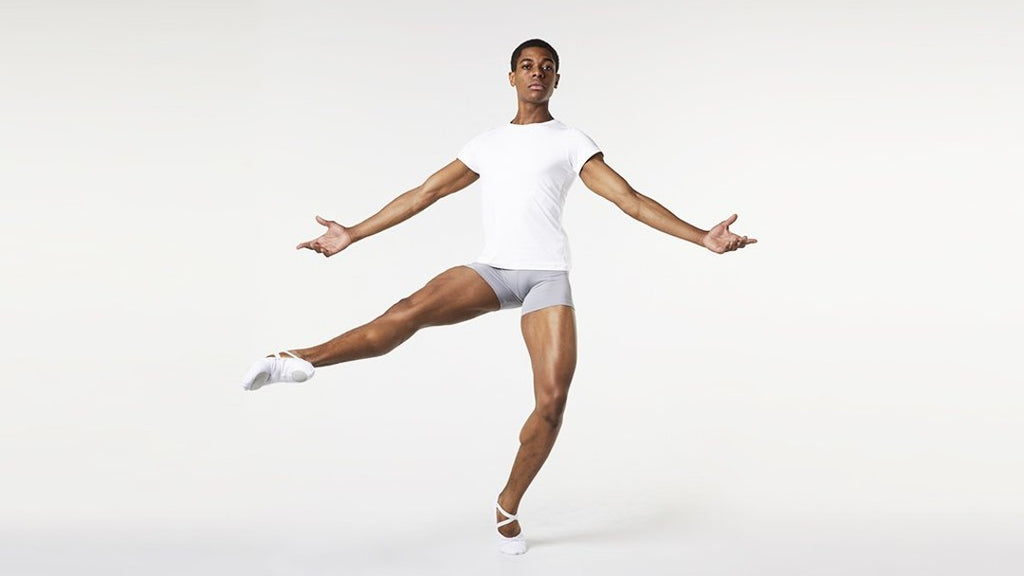This photograph captures a young African-American male ballet dancer in a minimalist white room, exuding a sense of effortless grace and strength. The dancer, in his twenties, stands poised on his left leg, balanced on the tip of his toes, with his right leg extended straight out to the left, foot pointed and curved. His arms are gracefully outstretched to the sides, with palms slightly facing upward. He dons a plain white t-shirt and snug gray or blue boxer briefs, accentuating his well-toned, muscular legs and arms. White ballet slippers with gray pads on the soles complete his attire. He gazes slightly above the camera with a composed and natural expression, reflecting the ease with which he performs this demanding pose. The background is entirely white, offering no visual distractions and allowing the viewer’s focus to remain solely on the dancer’s impressive form and technique. Shadows on the floor hint at the professional, artistic nature of the image, captured in a horizontal, borderless frame.